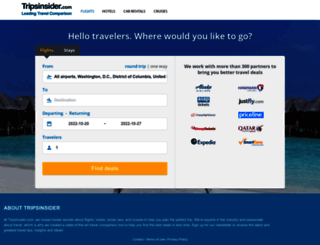This image is a screenshot from the TripInsider website, heavily blurred and rendered with an inch-wide white border. Positioned near the top left corner in black, bold text is the site’s name, TripInsider.com. Directly below it are three unreadable words in blue, accompanied by an adjacent blue word followed by three indistinct black words. The rest of the layout features a dark blue background.

A scenic, yet partially obscured image spans the screenshot's midsection, displaying faint glimpses of the sky, buildings, and water on both sides, along with sand. Overlaid at the top of the image, the text reads, "Hello Traverse. Where would you like to go?" in white.

Dominating the image is a light blue pop-up tab. At the top left of this pop-up are two gray tabs with illegible orange and white text, respectively. Below these is blue text, followed by a long white rectangle containing black text, succeeded again by blue text and another long white rectangle.

Continuing down the pop-up tab, two blue words precede a sequence of three rectangles interspersed with blue text, followed by another long yellow rectangular button stating, "Find Deals" in white.

On the right, there are two lines of blurred information, beneath which are icons representing five different stores. At the bottom left of the pop-up, the text "About Transparency" appears, with three additional unreadable lines of information below it.